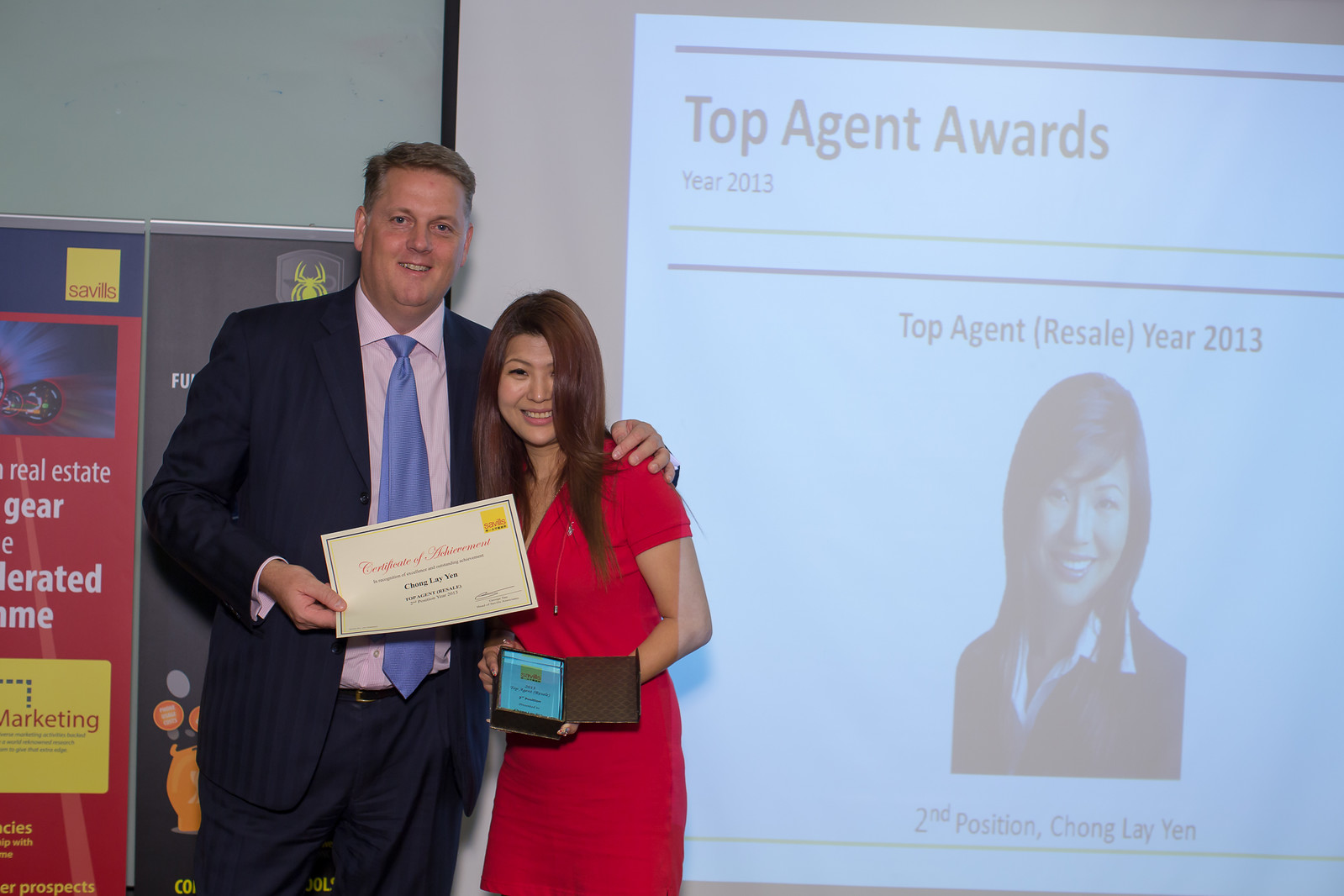The image depicts a celebratory moment on what appears to be a stage, where a tall Caucasian man with blonde hair, dressed in a black suit and blue tie, has his arm around a shorter Asian woman with caramel-colored skin and long dark brown hair. Both are smiling happily. The woman is wearing a short-sleeve red dress and holding an award or certificate, while the man holds a piece of paper, possibly a congratulatory document. Behind them, a screen is prominently displayed with the text "Top Agent Awards Year 2013" and "Top Agent Resale Year 2013," featuring the woman's image and announcing her second position with the name "Chong Lai Yen." The backdrop also shows some marketing signs and a white wall, enhancing the formal atmosphere of this award ceremony.